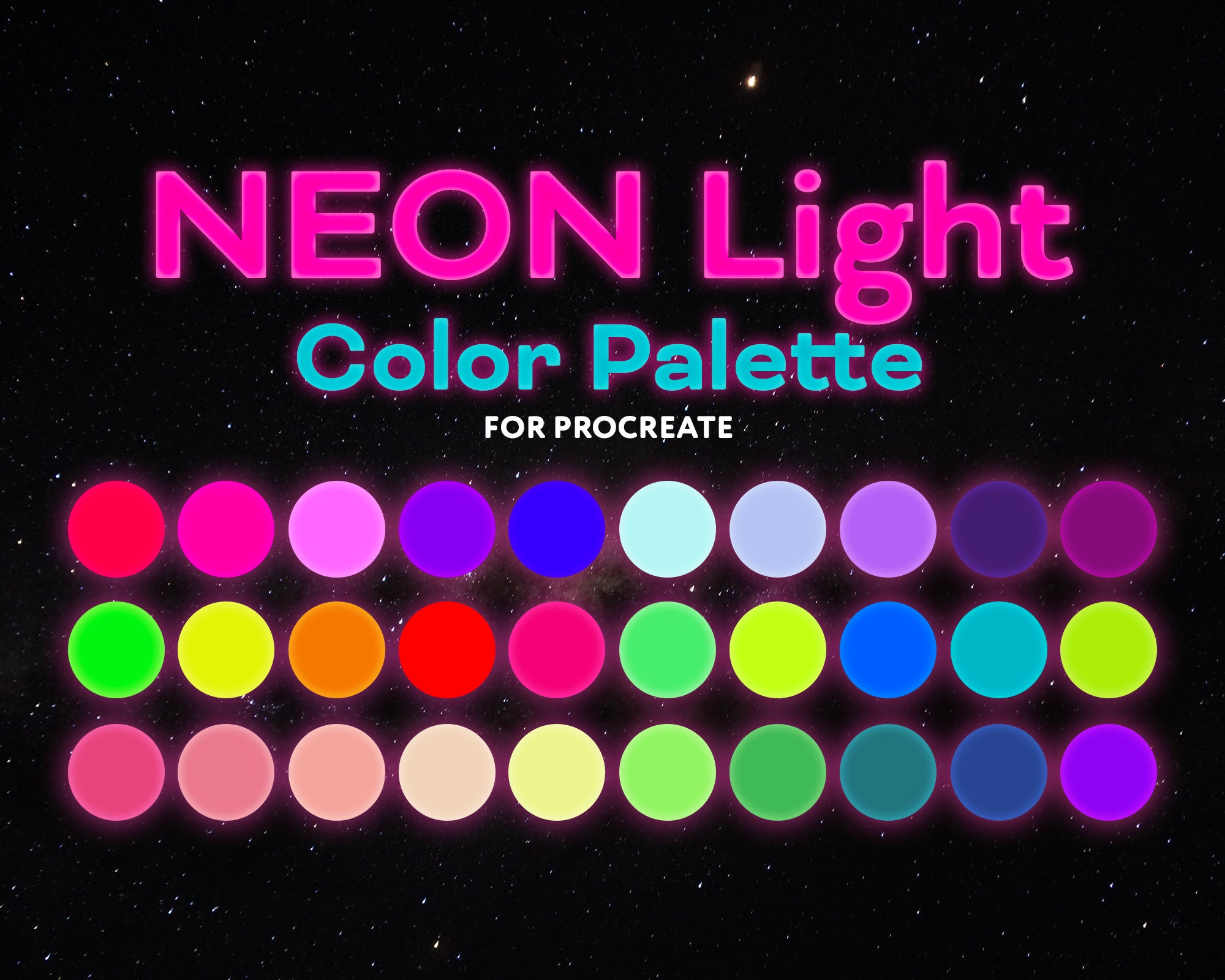This image features a vibrant, neon-themed color palette against a black background speckled with small white dots, resembling a night sky with stars. Dominating the top of the image, the words "Neon Light" are displayed in large, bold pink letters. Below this, "Color Palette" is written in light blue lettering, followed by "For Procreate" in smaller white letters. The main focus of the image is three rows of multicolored circles, each row containing ten circles. These circles exhibit a wide array of bright neon colors, including shades of red, pink, purple, blue, light green, yellow, beige, rose, and peach. This serves as a detailed illustration of the variety of vibrant colors available for Procreate.